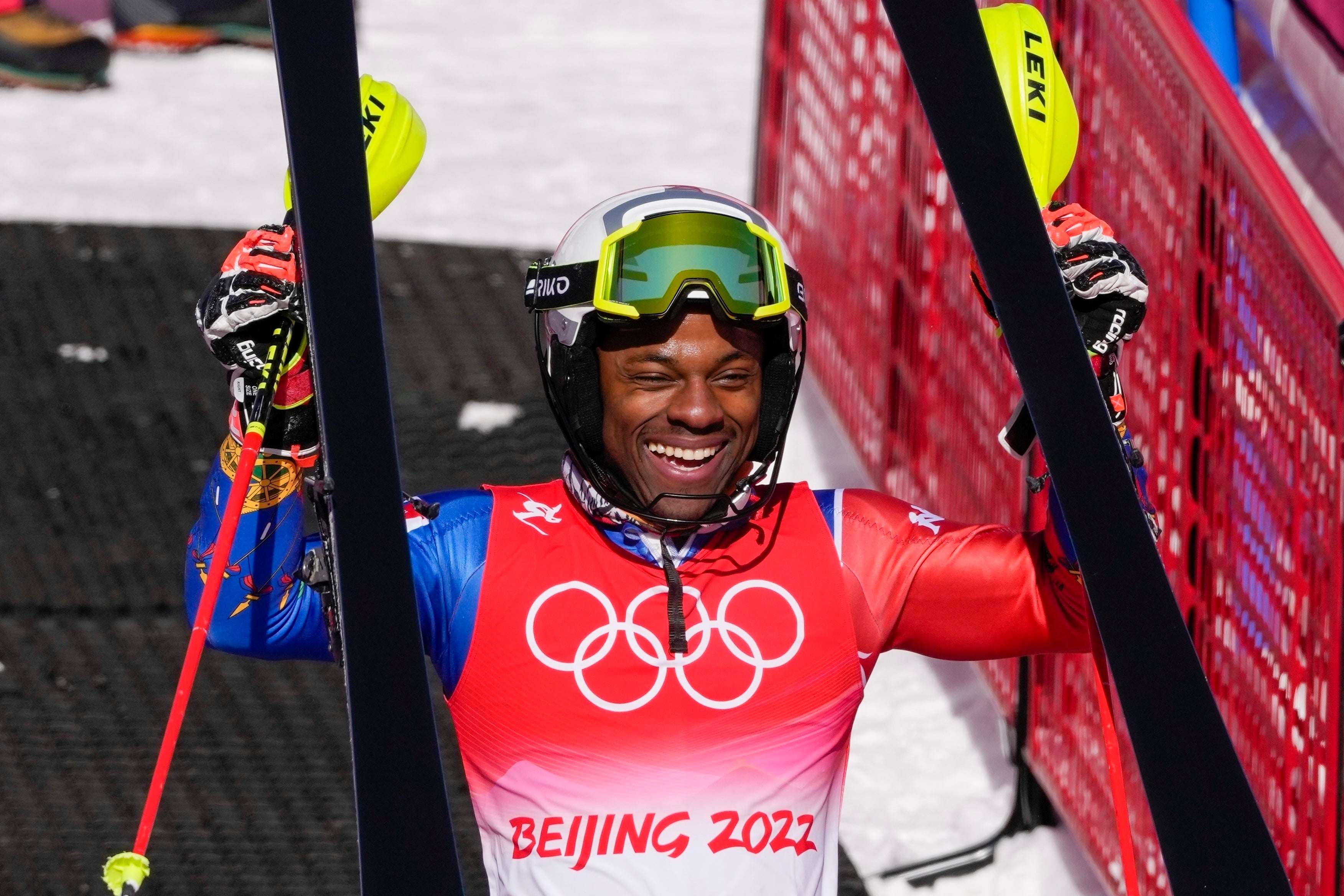The image captures a jubilant African-American skier at the Beijing 2022 Winter Olympics, standing triumphantly on a snow-covered ramp. He is adorned in a vibrant outfit with a predominantly red vest featuring the Olympic rings in white and "Beijing 2022" inscribed below. His right sleeve is blue while the left is red, each matching the overall color scheme. A white silhouette of a skier is visible on his top left shoulder. He wears a white helmet with yellow ski goggles perched above, allowing his beaming smile to shine through—a clear indication of his delight, possibly after a successful run or win. In both hands, he holds his skis aloft; the skis feature black bottoms and brightly colored red and yellow handles. His black and red gloves, with hints of white, complement his gear. Nearby, an orange mesh fence is visible, demarcating the spectator area from the track. The snow-covered background and black matting at the bottom of the slope suggest he is at the conclusion of his event, basking in his accomplishment.